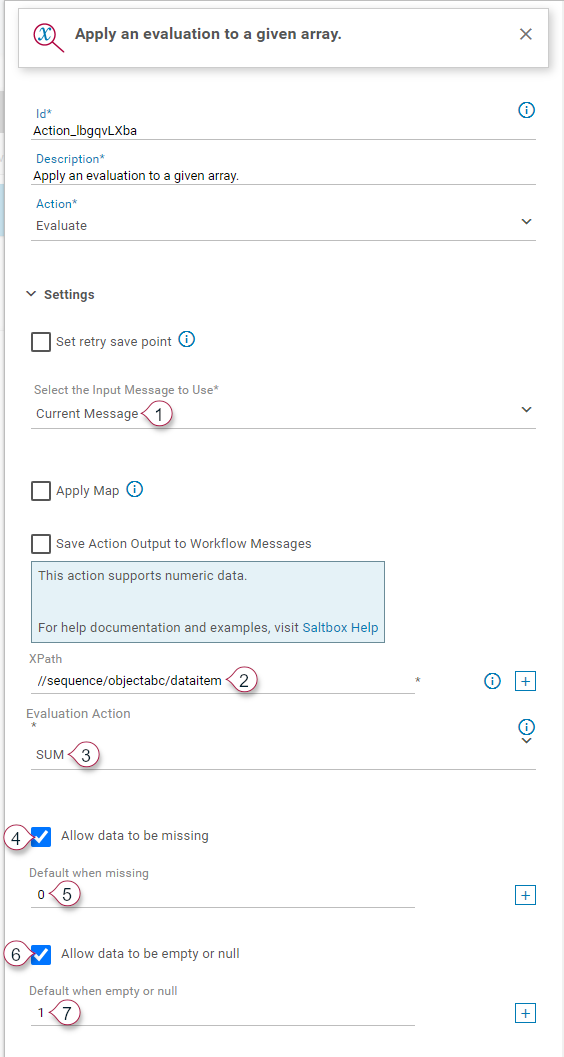The image depicts a detailed configuration page primarily for setting up an evaluation on a given array. At the top of the page, there is a search box labeled "Apply an evaluation to a given array." Below this, the page lists various fields and inputs: 

- "ID *" with the value "action_LBGQVLXBA".
- "Description *" with the text "Apply an evaluation to a given array."
- "Action *" with the value "Evaluate" and a drop-down arrow beside it.

Following these fields is the section labeled "Settings," which includes an unchecked box labeled "Set retry save point" with an information icon (i) next to it.

Further down, under the heading "Select the input message to use *" is the option "Current message" with the number 1 in a circle next to it. Below this is the "Apply map" option. The next line reads "Save action output to workflow messages," accompanied by a note stating, "This action supports numeric data. For help documentation and examples, visit Saltbox help."

The section then continues with "XPath Evaluation/Action":

- "Allow data to be missing" with a blue square icon containing a white checkmark and the number 4 beside it.
- "Default when missing," showing a 0 followed by the number 5 in a circle.
- "Allow data to be empty or null" next to another blue square with a white check mark and the number 6.
- "Default when empty or null" with a 0 and the number 7 in a circle.

The detailed text helps illustrate the step-by-step configuration process for the evaluation action on the page.